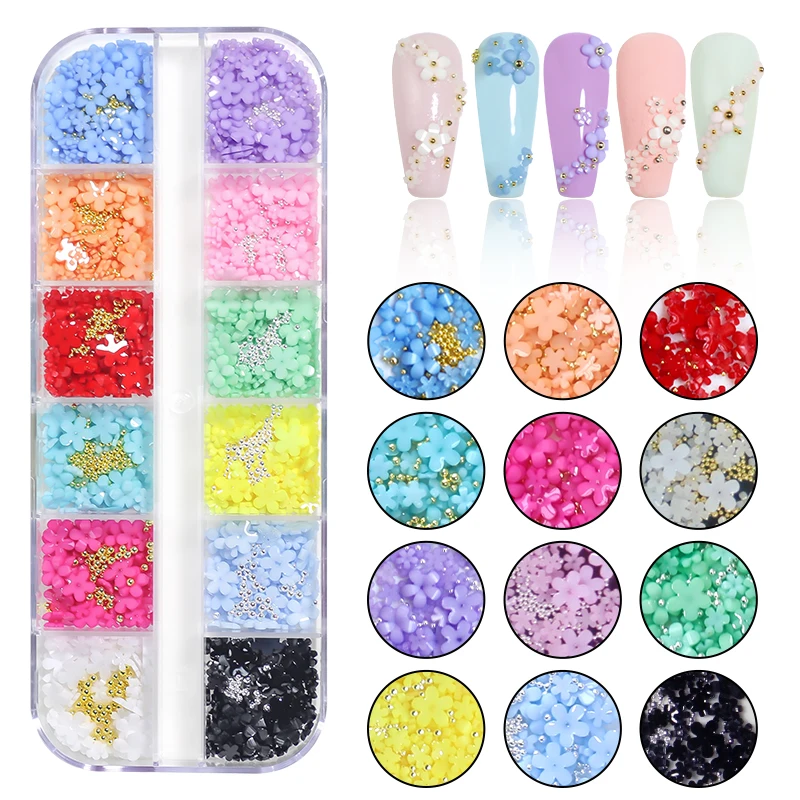This image is an advertisement collage showcasing a bead kit specifically designed for nail art. The central element is a vertically arranged transparent container with 12 partitions, each filled with small flower-shaped beads in various colors, including blue, orange, red, light blue, pink, white, purple, green, yellow, black, hot pink, and pale blue. Each vibrant bead compartment, resembling an ice tray, neatly organizes the flowers, with some beads featuring tiny yellow centers. To the right of this container, circular close-ups provide an enlarged view of the detailed flower beads, highlighting their intricate design and vibrant colors, which include variants of blue, pink, green, and yellow. Above these close-ups, a set of five artificial nails decorated with these flower beads is displayed, showcasing possible nail art designs. The nails come in colors such as white, blue, purple, pink, and green, each either matching the bead colors or featuring white floral accents.